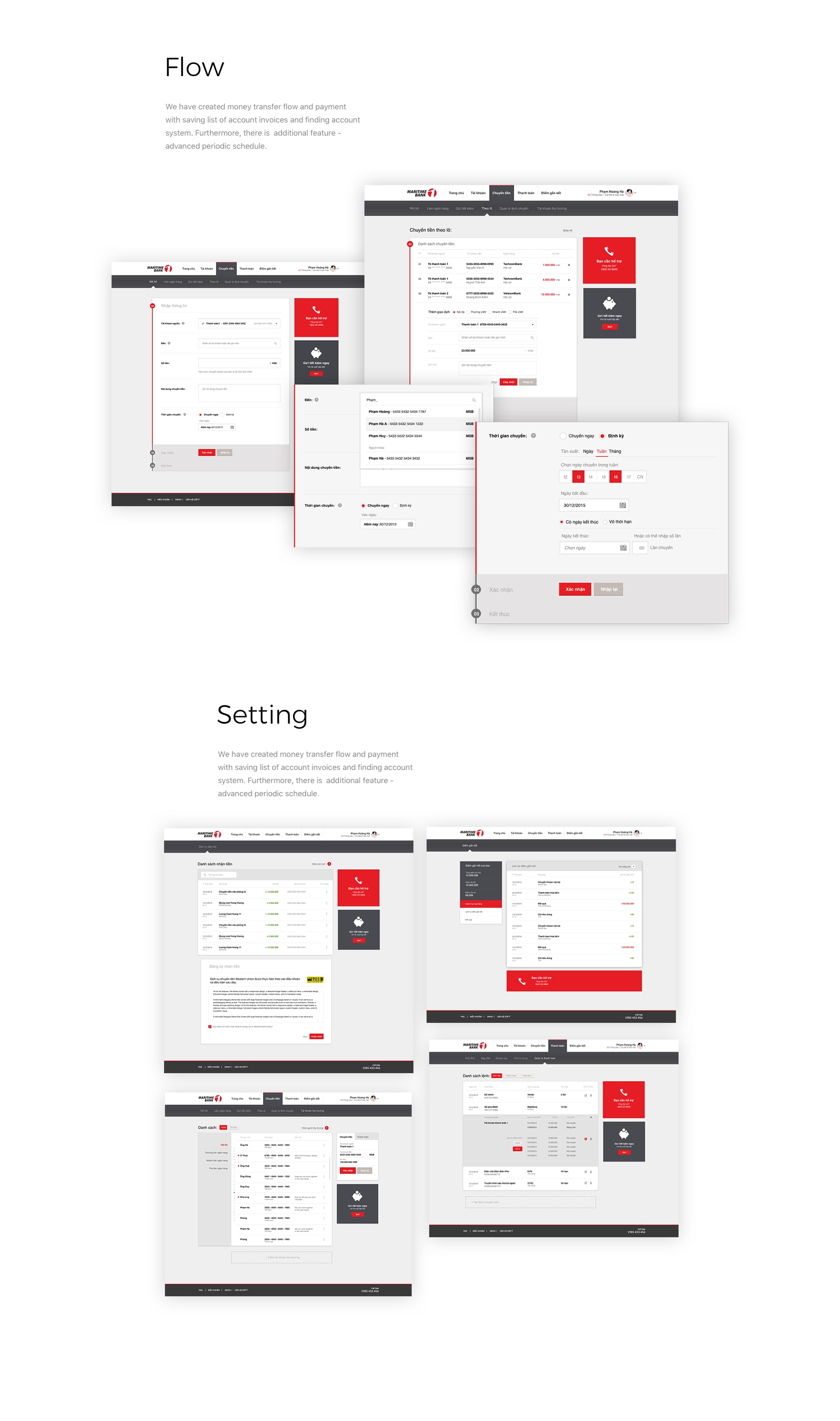The image is divided into two sections, one above the other. 

In the top section, there are four square-shaped cascading windows set against a light gray background with red and black color elements. All windows feature text that's too small to read. In the top left corner, the word "Flow" is visible, followed by four lines of black text, which are also too small to decipher. Among the four windows, two feature black borders at the top and bottom with unreadable text and contain red and black square elements. The other two windows are smaller and lack the black borders.

The bottom section mirrors the top with another set of four equally-sized square windows, each bordered by black lines at the top and bottom and containing unreadable text. The word "Setting" appears above this section, along with four lines of black text, similarly too small to read.